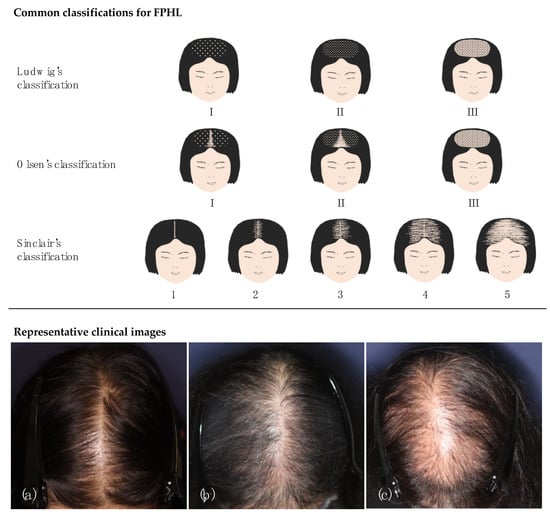The image appears to be a detailed page from a clinical textbook or study on Female Pattern Hair Loss (FPHL), particularly showcasing various classification systems used to categorize the stages of FPHL. The title at the top reads "Common Classifications for FPHL". On the left side, we see the headers for three different classification systems: Ludwig's classification at the top, followed by Olsen's classification, and then Sinclair's classification. 

The page includes a series of computer-generated images depicting patterns of hair thinning in an Asian woman, arranged in three rows. The first two rows each show three images across, while the third row shows five images. These images illustrate the progressive stages of balding according to each classification system. Below these rows, there's a black horizontal line separating the images from another section.

In the lower section, labeled "Representative Clinical Images," there are three photographs (A, B, and C) of the top of a woman’s head with black hair, demonstrating the clinical appearance of FPHL. Image A shows a head with mild thinning, image B illustrates more pronounced thinning, and image C shows severe hair loss with significant balding areas.

The color scheme of the page predominantly features light brown, white, and black tones, contributing to the clarity and emphasis on the visual information presented.